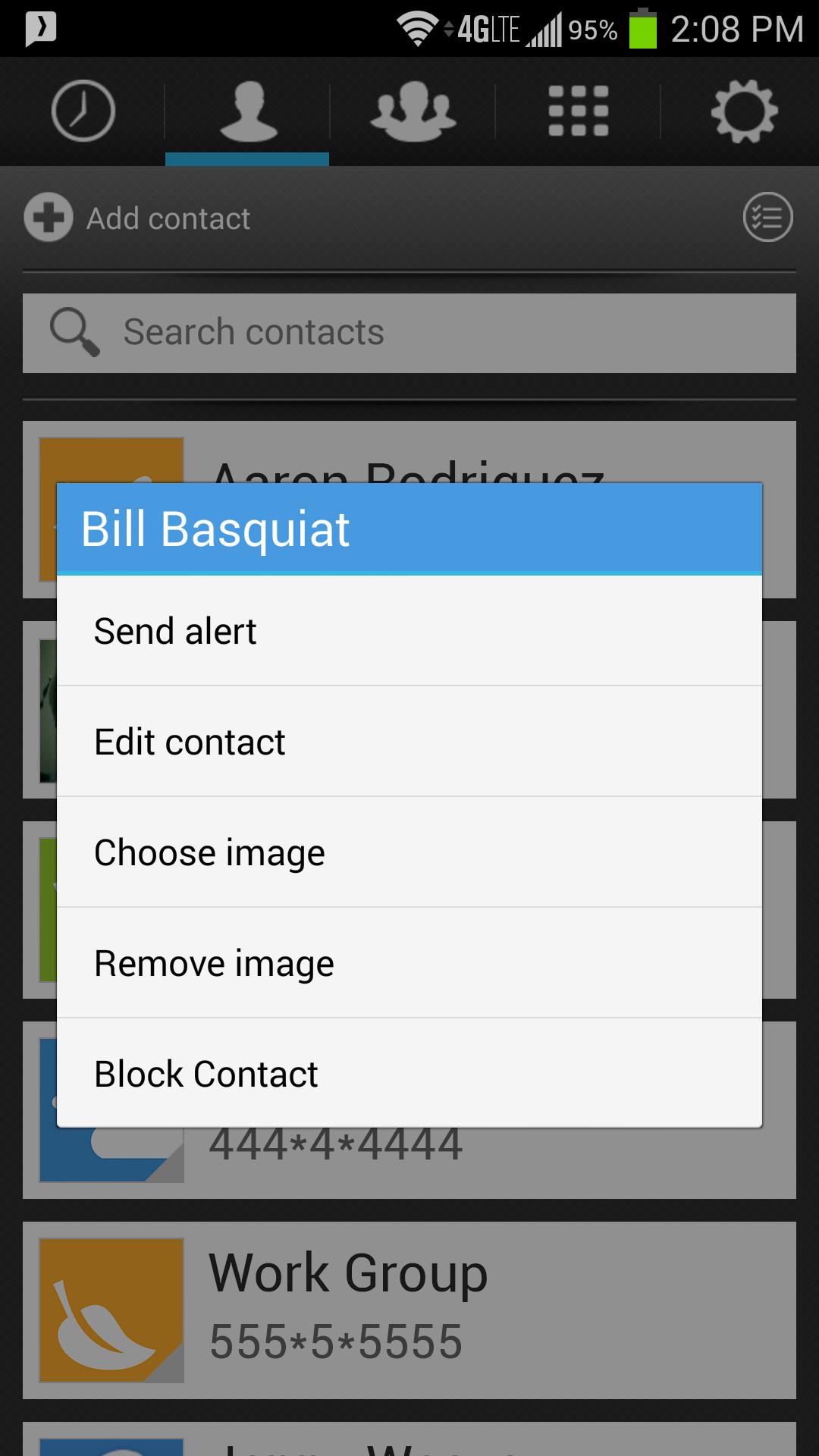This is a detailed screenshot taken on a mobile phone screen. In the upper right-hand corner, the time displays as 2:08 PM. Positioned to the left of the time is the battery percentage indicator showing 95%, with icons for cell phone signal strength and Wi-Fi coverage strength adjacent to it, indicating that the device is using a 4G LTE service.

In the upper left-hand corner of the screen, there is a small icon of a box with an arrow pointing to the right. Below this icon, a row of four icons is arranged from left to right, each representing different functions: a clock icon, a contact icon, a multiple contacts icon, and a menu/settings icon.

The screenshot reveals that the user currently has a single contact open, as indicated by the blue bar under the single contact icon. The contact displayed is "Bill Basquiat." Below the contact name, there are several options available for interaction: "Send Alert," "Edit Contact," "Choose Image," "Remove Image," and "Block Contact."

This display appears as a pop-up over the user's contact list, which is partially visible in the background, showing additional contacts such as "Aaron Rodriguez" and "Work Group." The pop-up obscures part of the contacts page but provides the necessary options for managing the selected contact, Bill Basquiat.